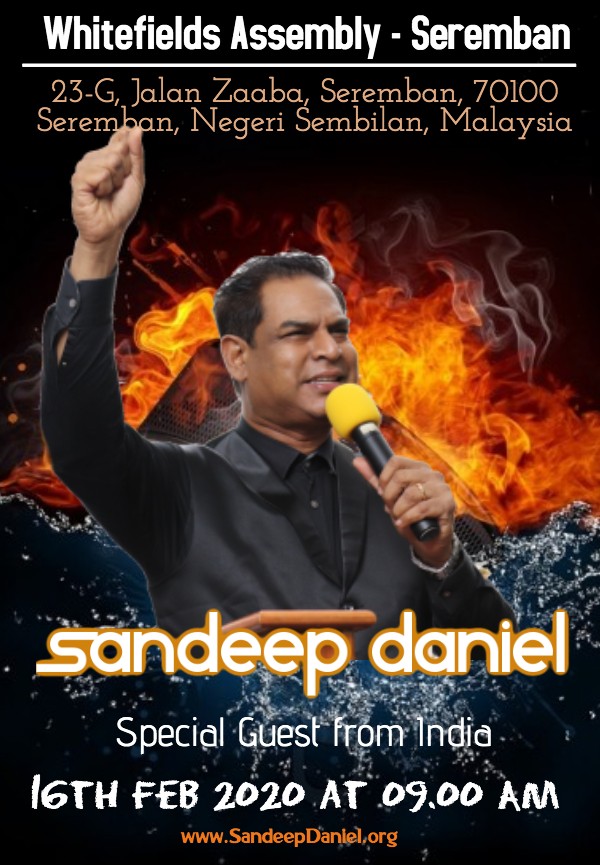The poster features a black background with dramatic, photoshopped flames in the middle. At the center is a dark-skinned man from India with bronze complexion and short black hair, dressed in a black suit. He is holding a microphone in his left hand, and his right hand is raised in a fist. At the top of the poster, the text reads "Whitefields Assembly, Seremban, 23rd-G, Jalan Zaba, Seremban 70100, Seremban, Negeri Sembilan, Malaysia." Below the man, it announces "Sandeep Daniel, Special Guest from India, 16th February 2020 at 9am." At the very bottom, the web address "www.sandeepdaniel.org" is displayed.